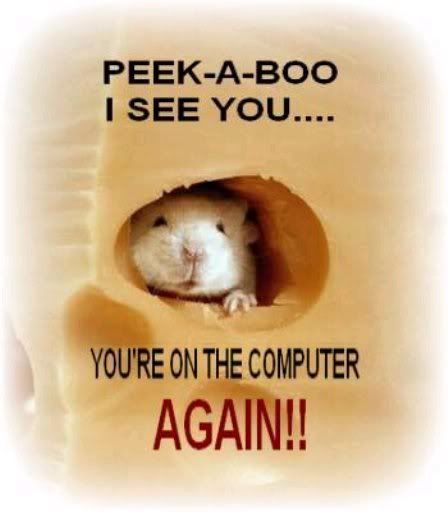This humorous meme features a light grayish PhotoBucket watermark prominently in the center, featuring the PhotoBucket logo on the left. At the top of the image, the text "PEEKABOO I SEE YOU" is displayed in large, all-caps black font. Below this, a white mouse or rat with its mouth slightly open is peeking out from a tunnel it has dug in a yellow cube of cheese. The text "YOU'RE ON THE COMPUTER AGAIN!!" is placed below the mouse in large, black capital letters, emphasizing the joke's playful tone. Additionally, a banner beneath the watermark reads, "Protect more of your memories for less!" with a couple of exclamation points for emphasis. The image's elements, such as the colorful cheese and the engaging text, make it an apt and fun reminder about time spent on computers, all in keeping with the meme-style humor.